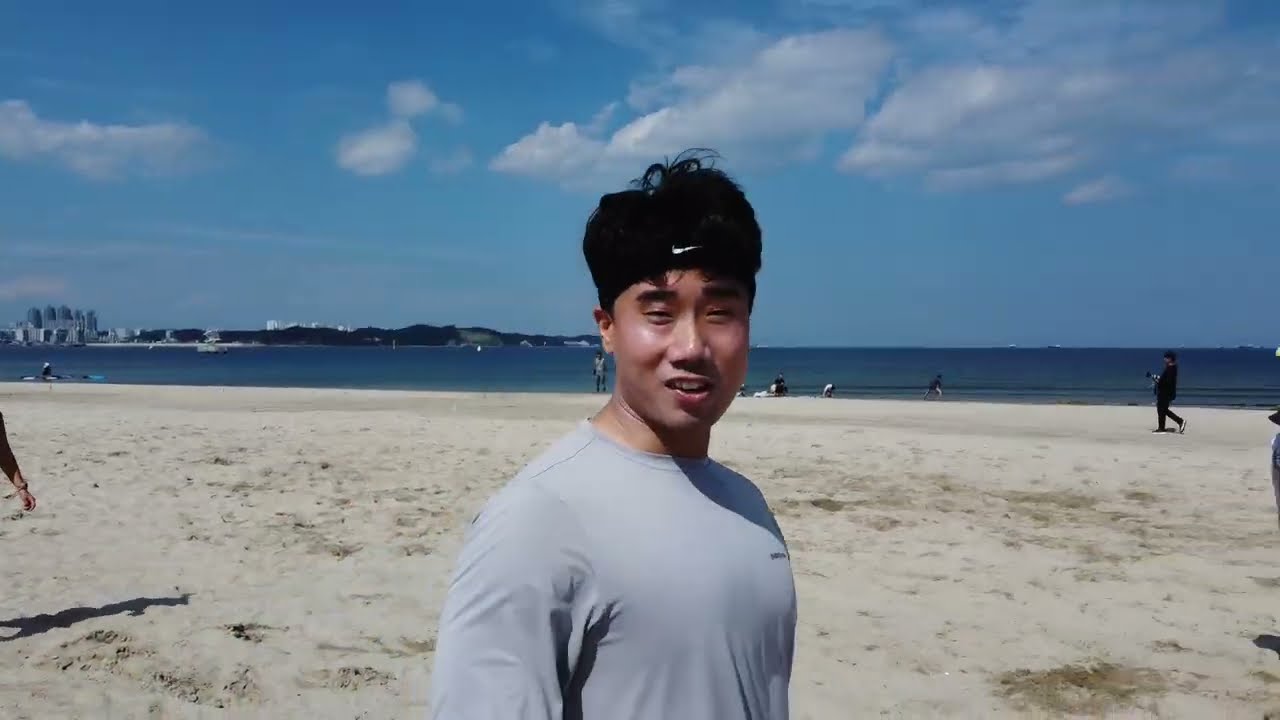The image captures an Asian man with black hair, wearing a gray long-sleeve shirt and a black Nike headband, smiling as he takes a selfie on a sunny beach. The beach, covered in brownish sand with occasional washed-up seaweed, stretches behind him where several people can be seen walking, playing, and casting shadows. The sky is blue with high white clouds, and the calm, blue water extends to the horizon. In the distance, on the left side of the image, there's an island or another piece of land, possibly with some buildings or hotels. Near the shore, a small boat is visible, along with people enjoying the water at the shoreline. Additionally, there are ships or other objects faintly visible on the distant horizon.